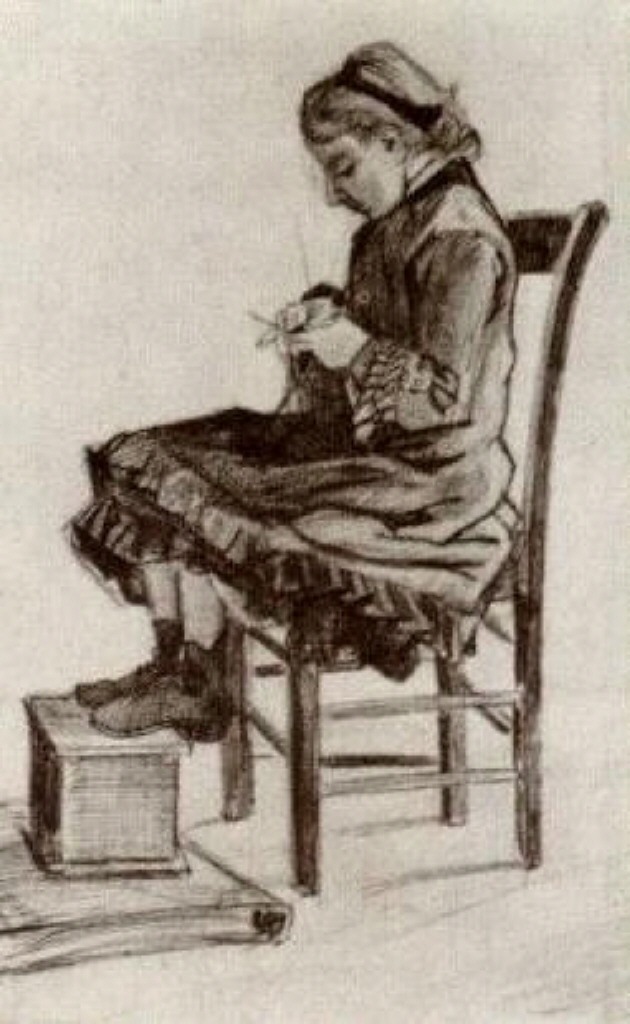This is a vertical, rectangular pencil or charcoal drawing depicting a young woman or girl seated in profile on a high-backed wooden chair, facing left. She has her feet resting on a small wooden footstool, which is elevated atop a book. She appears to be engaged in knitting or sewing, attentively looking down at her hands. The illustration provides minimalistic details, emphasizing a sparse and aged aesthetic with sepia tones reminiscent of an old photograph. The girl is wearing a dress with frills at the bottom and sleeves, and black boots on her feet. Her hair is neatly tied up, adorned with a ribbon or bow, suggesting a modest but careful arrangement. The background remains unembellished, enhancing the focus on the serene and meticulous figure absorbed in her task.